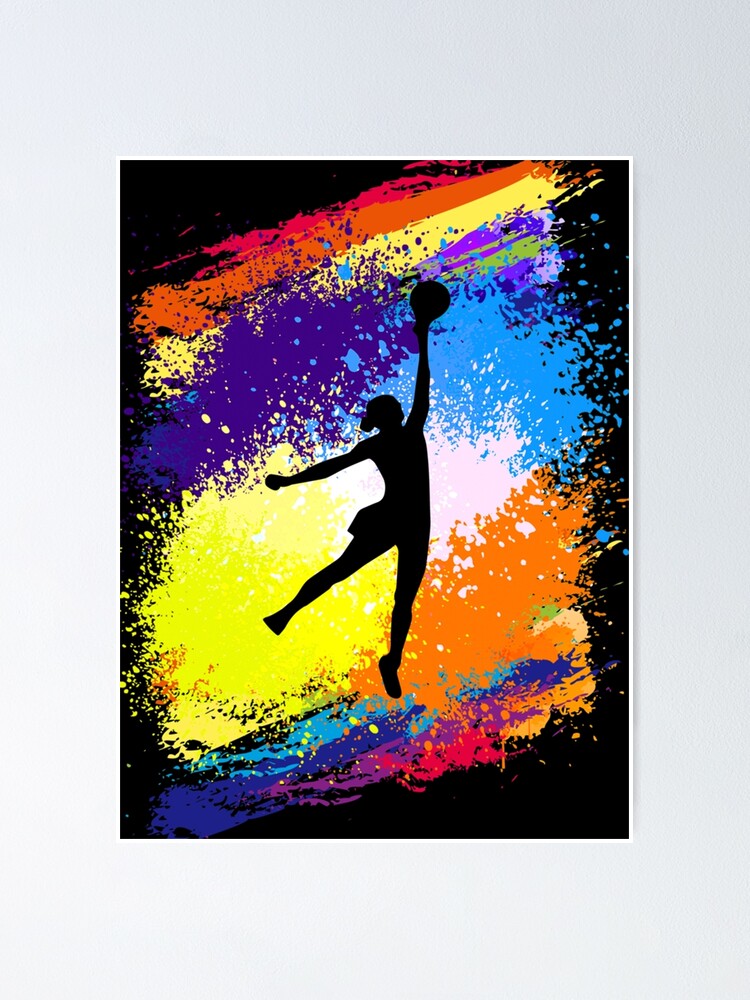In this image, we see a striking design featuring a complete black silhouette of a person in an athletic pose reminiscent of the Air Jordan logo. The figure’s right leg is firmly planted on the ground, while the left leg and left arm are artistically extended out to the side. The right arm is raised high, gripping a ball, and the head is depicted as a simple circular shape. Surrounding this dynamic silhouette is a vibrant, colorful backdrop featuring a series of hues that blend seamlessly together. The colors transition from blue, purple, and pink at the base, to orange and yellow, and then white at the very center, before shifting to light blue, purple, light yellow, orange, and pink towards the top. Adding to the visual impact are splash-like effects that accentuate the colorful background. The outermost layer of the image is a deep, solid black, providing a stark contrast to the vivid spectrum of colors and highlighting the boldness of the silhouetted figure.